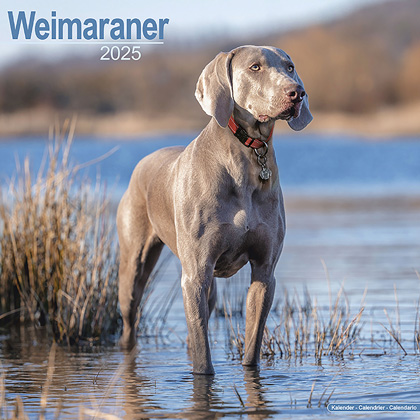The front cover of this 2024 calendar highlights a young Weimaraner, likely around six months old, as its main focus. The dog is positioned centrally, appearing to either stare directly at the viewer or off into the distance. It is predominantly brown with big floppy ears that are a lighter shade of brown, hazel eyes, and a black nose. The Weimaraner is lying on what seems to be a log, surrounded by stick branches protruding towards the lower left corner. The background is a blurry mix of brownish-gray hues, making it difficult to ascertain the exact setting. The dog is also sporting a brown collar with a buckle. In the upper left-hand corner of the cover, the word "Weimaraner" is displayed in white letters with a gray horizontal line underneath, followed by the year "2024" in gray numbers.